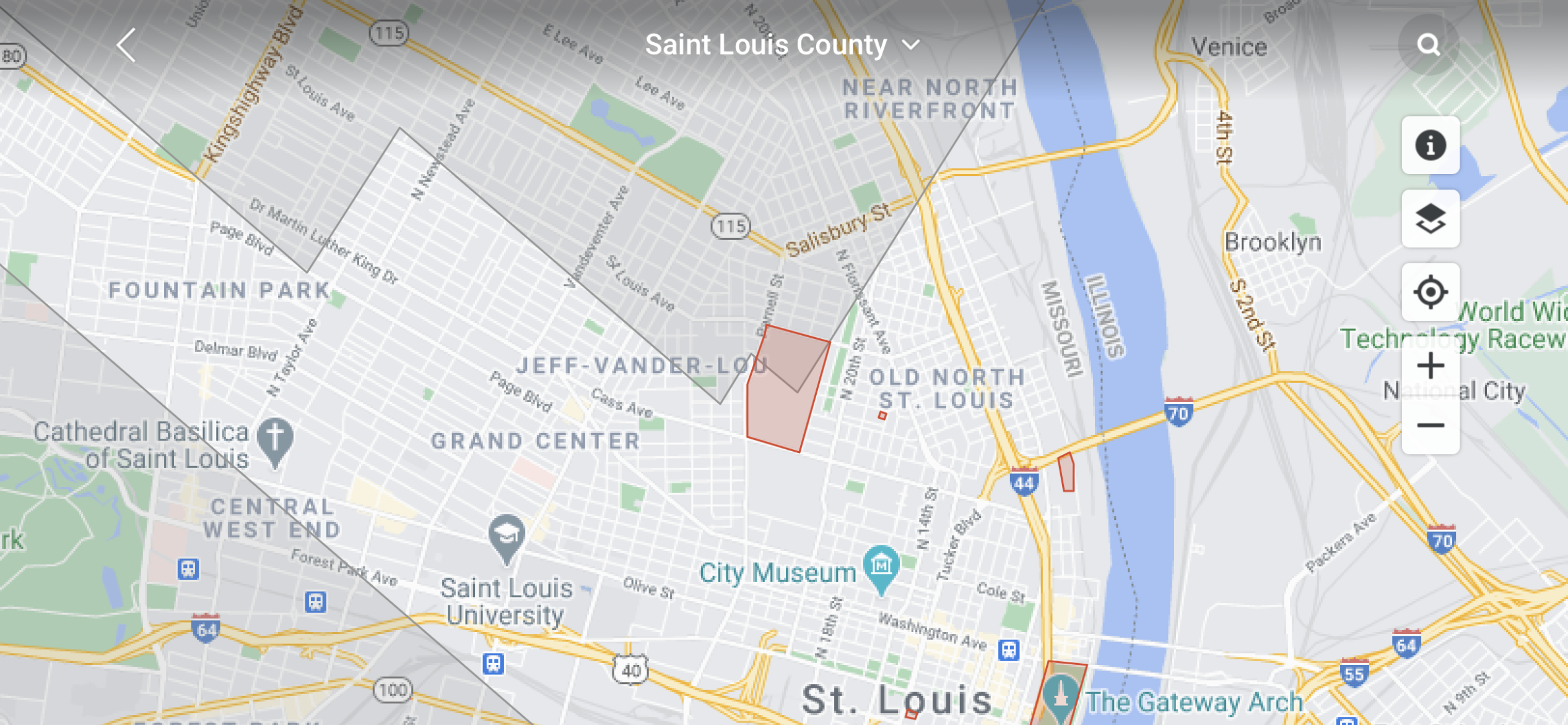The horizontally aligned, rectangular image is a detailed city map of St. Louis County, likely a screenshot from a GPS map on a cell phone, such as Google Maps or Waze. At the top center, in small white letters, it reads "St. Louis County" with a down arrow. In the upper left corner, there's a sideways V pointing toward a left arrow, and in the upper right corner, a small circle with a stem representing the search function. Vertically aligned icons appear on the right-hand side, including an 'I' for information, a square on top of another square, a compass, and a plus-minus sign.

The map primarily depicts gray areas, interspersed with green sections, red sections, and blue areas. A prominent vertical blue line represents the Mississippi River, dividing Illinois on one side and Missouri on the other. Significant highways include Route 64 running horizontally across the bottom, Route 44 extending from the bottom to the top, and Route 70 branching off. In the lower right corner, highways 55 and 64 intersect.

Landmarks and cities identified on the map include St. Louis at the very bottom, Old North St. Louis in the center, and Near North Riverfront at the top. Additional points of interest include Fountain Park, Cathedral Basilica of St. Louis, Central West End, the City Museum, and St. Louis University. An upside-down teardrop marks the location of the Gateway Arch. The major roads are highlighted in yellow, clearly labeled with their respective route numbers.